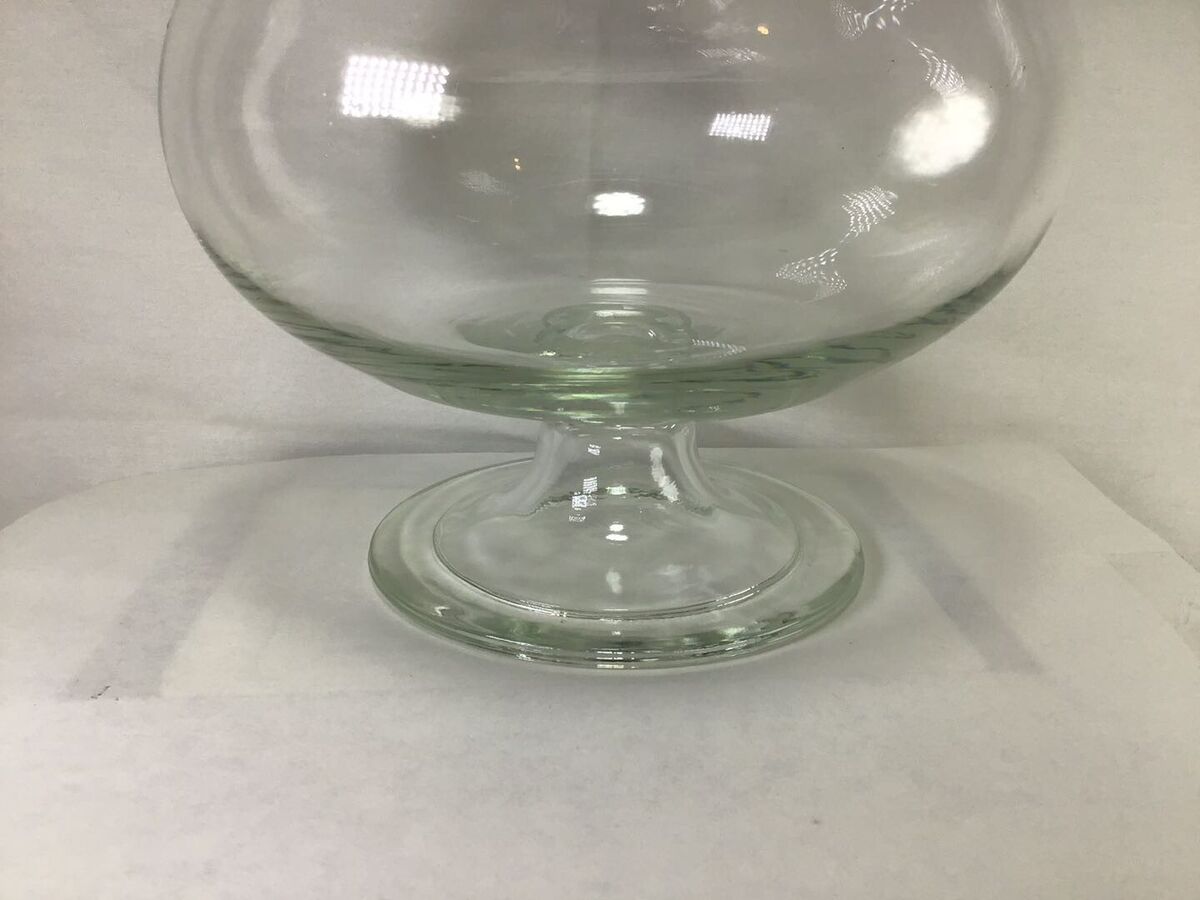The image depicts a close-up view of a clear glass goblet or bowl, prominently showcasing its design and the lighting effects around it. The glass is resting on a white surface, possibly a tablecloth or napkin, and the background is also white, adding to the minimalist setting. The goblet features a small, round base and a narrow stem that expands into a wide, empty bowl at the top. The glass appears to be thick, especially noticeable at the bottom of the bowl. Vertical dark lines or gray shadows flank the base, while reflections and highlights from the lighting create various light patterns on the glass surface. These reflections, resembling spotlights, add depth and dimension to the photograph. Despite the close-up nature of the image, which makes it difficult to gauge the exact size of the goblet, the detailed reflections and clean white background draw significant attention to the intricate features of the clear glass object.